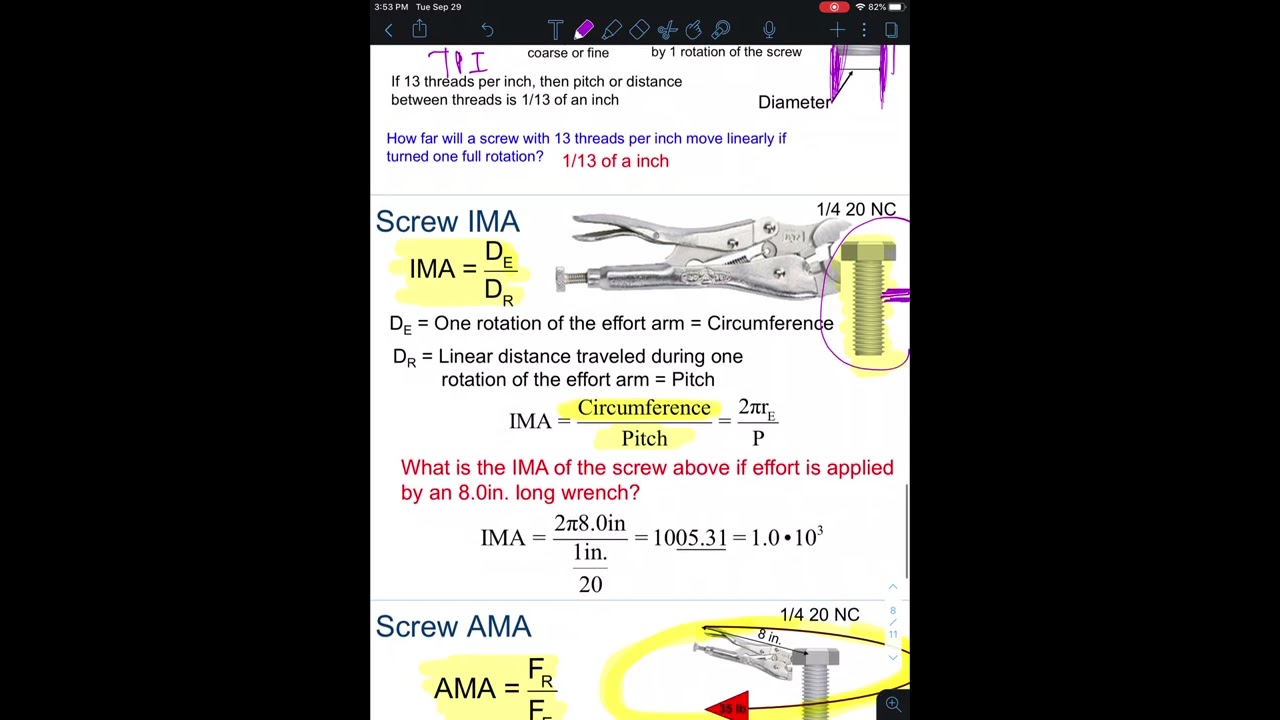The image is a screenshot from a mobile device, displaying a detailed presentation on mechanical concepts. It includes editing tools in a black bar with a blue outline at the top, and the device details indicate it's 3:53 PM on Tuesday, September 29th, with an 82% battery level. The presentation is divided into three sections:
1. The top section explains the relationship between thread pitch and screw rotation, stating "Coarse or fine by one rotation of the screw." With 13 threads per inch, the pitch is 1/13 of an inch. It asks, "How far will a screw with 13 threads per inch move linearly if turned one full rotation?" and answers in red, "1/13 of an inch." An illustration displays the term "diameter" with a black arrow and purple markings.
2. The middle section, titled "Screw IMA," highlights formulas and concepts related to the screw's Ideal Mechanical Advantage (IMA). Key equations include "IMA = D subscript E over D subscript R" and "IMA = circumference over pitch = 2πR subscript E over P." It features phrases like "D = one rotation of the effort arm equals circumference" and "DR = linear distance traveled during one rotation of the effort arm equals pitch." Additionally, the question "What is the IMA of the screw above if effort is applied by an 8.0 inch long wrench?" is presented with a worked-out solution: "IMA = 2π×8.0 inches / 1 inch × 1 inch / 20 = 1005.31 ≈ 10³."
3. The bottom section, titled "Screw AMA," introduces Actual Mechanical Advantage (AMA) and its corresponding formula: "AMA = F subscript over R divided by a capital F." It includes an illustration of an 8-inch wrench and a screw, alongside an equation demonstrating the AMA calculation.

The image conveys essential information about thread mechanics and the application of mechanical advantage principles, utilizing visual aids and detailed formulas.